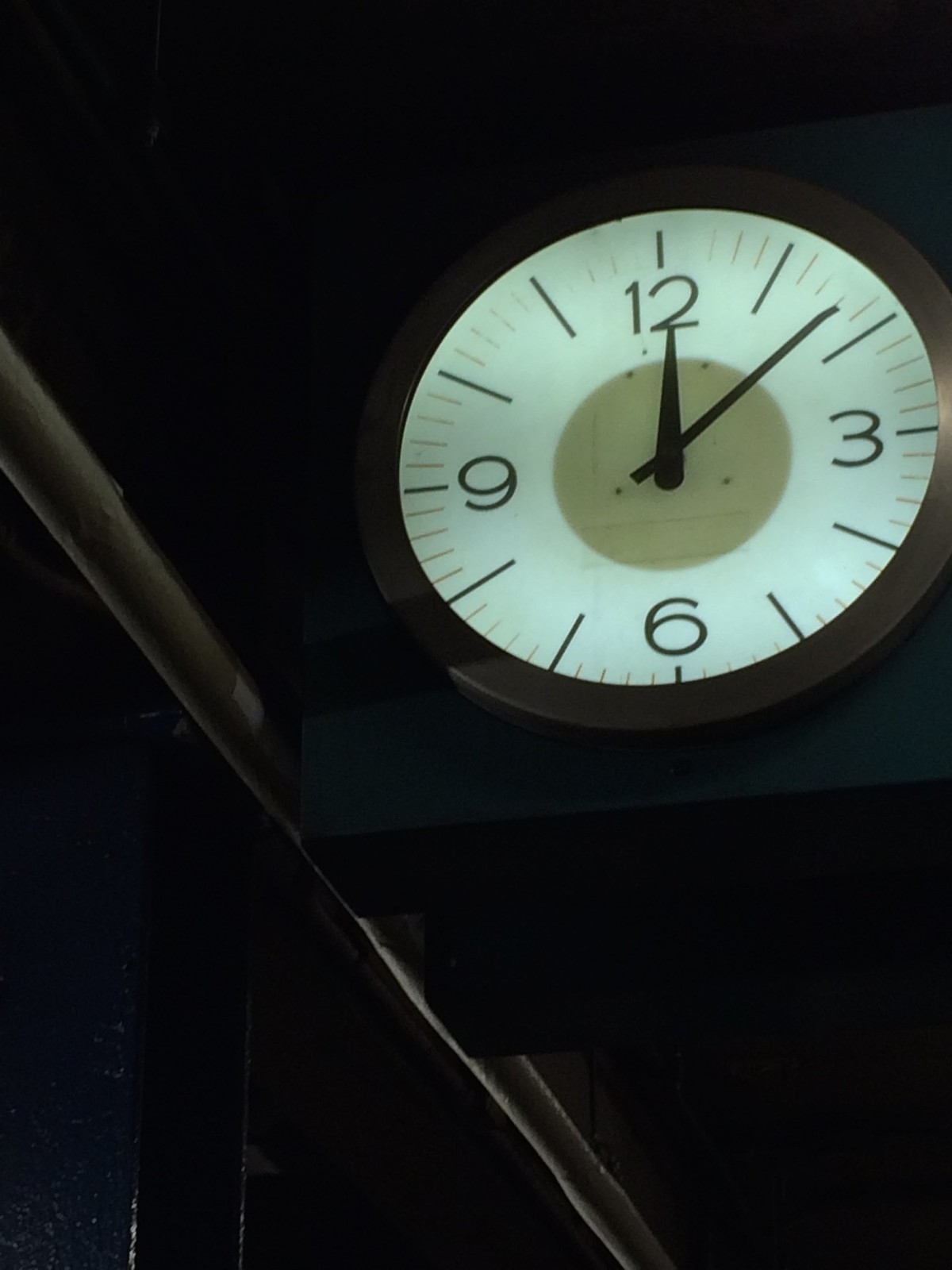This is a photograph capturing a dark and moody scene. Dominating the top right corner is a clock with a bold black outline. The clock's face is white, marked with the numbers 12 at the top, 3 at the right, 6 at the bottom, and 9 at the left, interspersed by simple dashes. The minute hand is approaching the 2, while the hour hand is fixed at 12, indicating the time is nearly 12:10. The clock is mounted on a stark black wall, contributing to the photograph's overall dark ambiance. To the side, a gray post subtly emerges, contrasting slightly with the surrounding black walls that frame the entire picture.